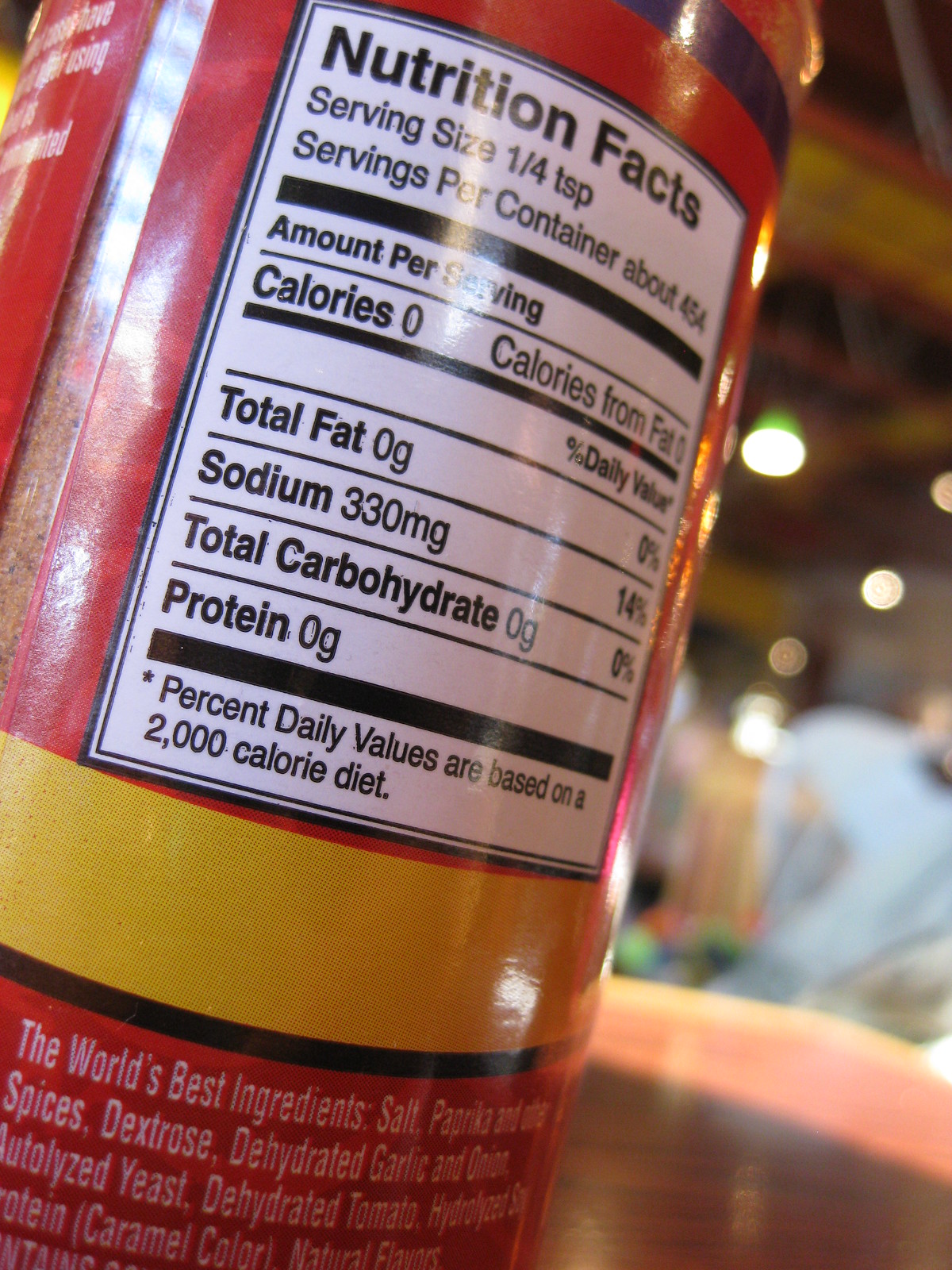The image in focus is a zoomed-in shot of the Nutrition Facts label on a plastic container, likely carrying a spice blend. The container, adorned with red and yellow accents and a yellow band, has a clear spot revealing orange powder inside. The serving size is listed as a quarter of a teaspoon, with approximately 454 servings per container. Nutritional details indicate that each serving contains zero calories, zero fat, and 330 milligrams of sodium, which is 14% of the daily value. The list of ingredients includes salt, paprika, spices, dextrose, dehydrated garlic and onion, autolyzed yeast, and dehydrated tomato. The background of the image is blurry, showing indistinct lights and a person in a light blue shirt. The container's label touts it as containing "the world's best ingredients," suggesting a rich, MSG-leaning flavor profile.